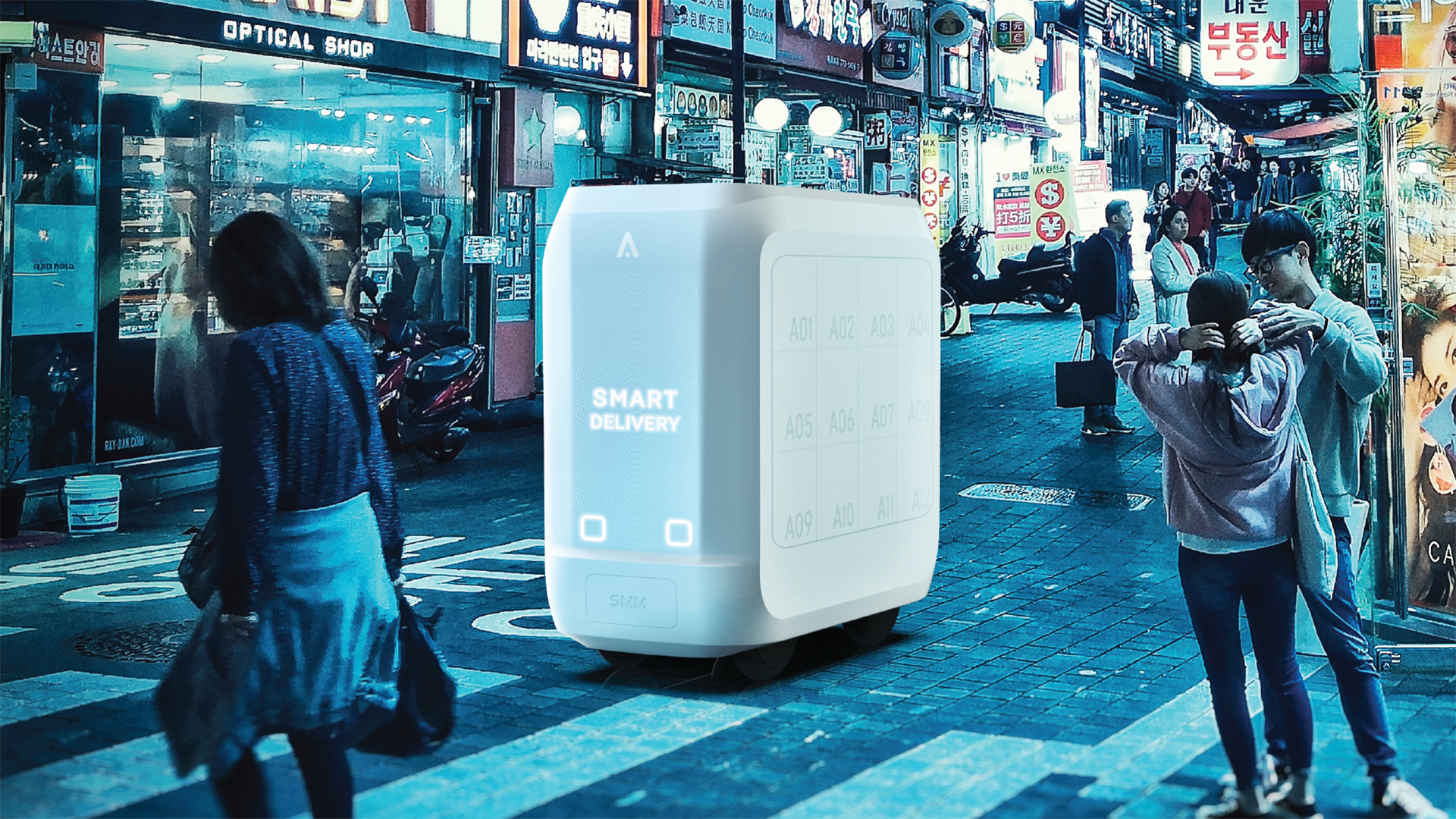The image depicts a bustling city street, likely set in a high-tech urban area in East Asia given the prevalence of signage in Korean. Dominating the center of the scene is a large, white, six-foot-tall delivery robot with four wheels. The robot features an illuminated "Smart Delivery" sign on its front and a side panel organized into a 3x4 grid of cubbies labeled A01 through A12, possibly for holding items awaiting delivery. The street is busy with people walking around, shopping, and engaging in conversation. Notably, a girl with her hand behind her head is talking to a man to the right of the robot. They are in front of an Optical Shop, among various other stores with vibrant signs. The road is marked with white lines, and the ambiance is one of lively urban activity.